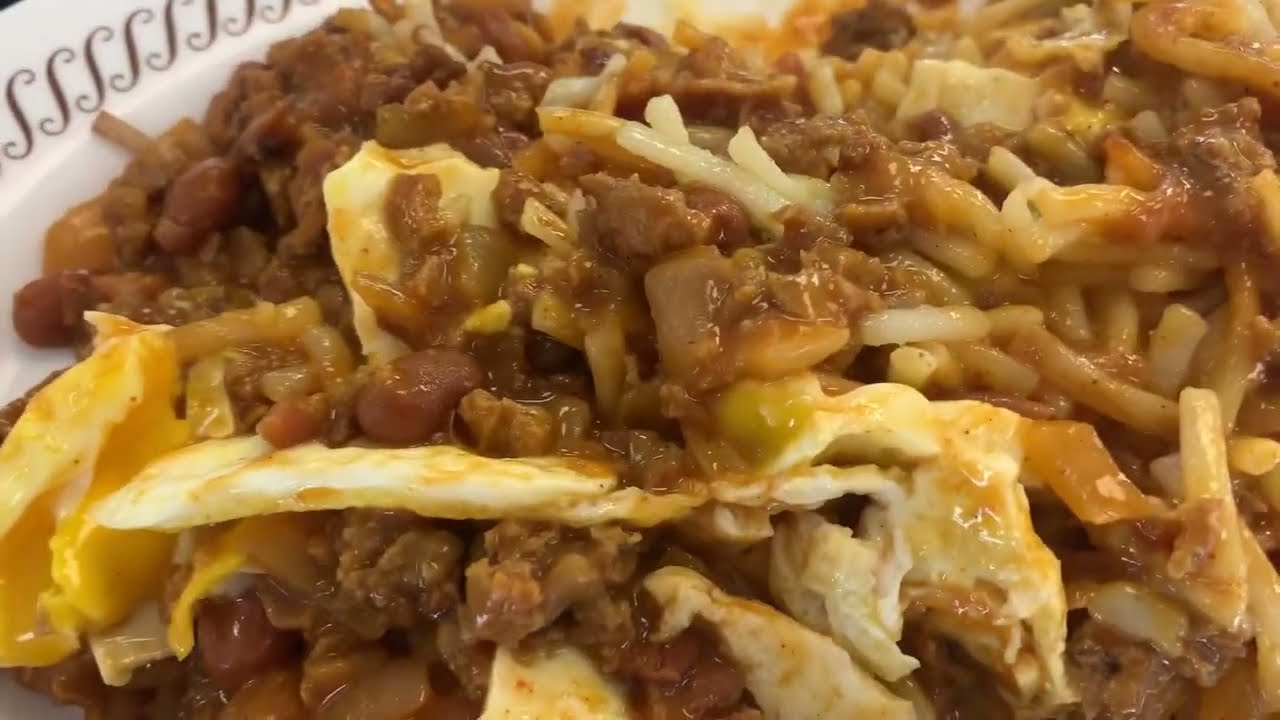This is a color photograph, taken in landscape orientation, depicting a close-up view of a dish of food, likely indoors. The image captures a detailed and vibrant depiction of a casserole-like dish in a white ceramic bowl adorned with a black scroll design along the rim. The dish appears to be a fusion of various ingredients, primarily featuring finely chopped, glistening brown ground beef. Interspersed within the meat are crushed soda crackers or bits of fried tortilla chips, which add texture and visual interest. Further enhancing the dish's complexity are small bits of white pasta or possibly rice, red chunks that could be tomatoes, and some brown beans. The overall color palette of the food ranges from browns and yellows to occasional hints of green and beige, likely from cheese, which could be mozzarella, topping the casserole. The extreme close-up shot fills the frame almost entirely, leaving just a glimpse of the bowl's ornate rim in the upper left-hand corner, emphasizing the intricate details and varied textures of the dish.